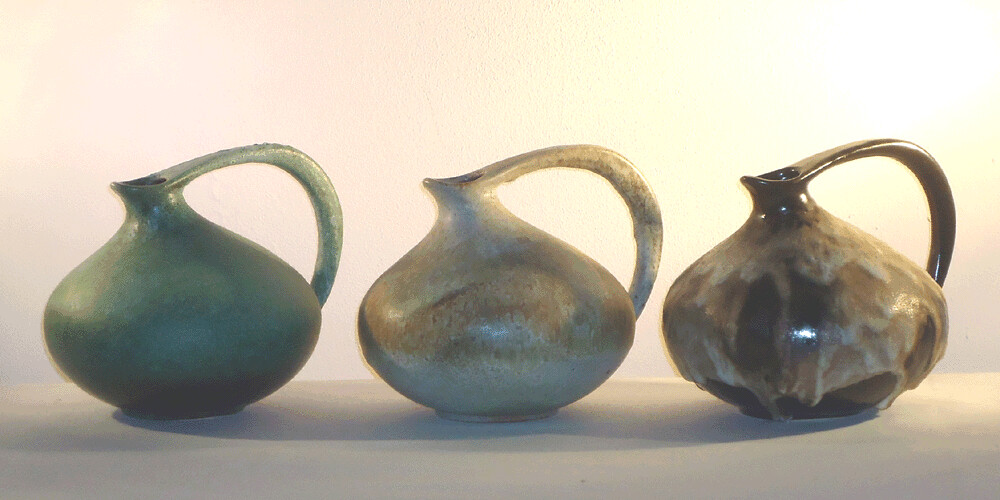The image features a set of three identically-shaped, pear-like vessels, each equipped with a large handle, seemingly intended as teapots or vases. The background transitions smoothly from a darker tan at the bottom to a lighter, peachy hue mixed with white and yellow towards the top, with hints of pink and gray interspersed, creating a soft, gradient effect. The leftmost vessel exhibits a green, slightly iridescent body, with a handle of a lighter green shade. The central vessel is predominantly slate gray, complimented by contrasting shades of brown and beige, giving it a more muted, earthy appearance. The rightmost vessel is vibrant and shiny, featuring a marbleized mix of dark brown, caramel, and off-white, with a brown handle accented by beige. These vessels rest on a beige floor that matches the background's palette, tied together by their similar yet distinct color schemes and pear-shaped designs.